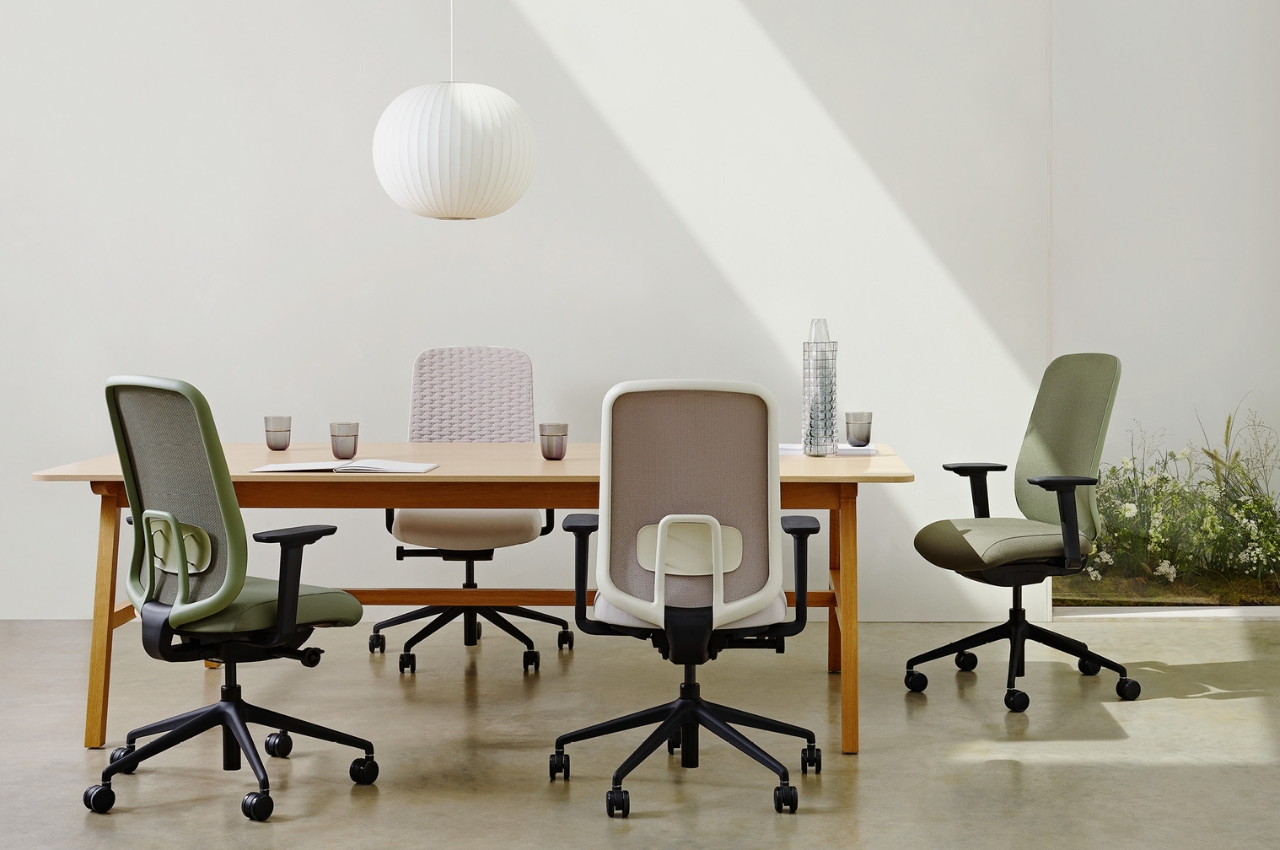This color photograph depicts a modern office conference room characterized by its light and airy ambiance. Dominating the image is a large light oak wooden table, occupying roughly two-thirds of the frame from the left to the middle. Surrounding the table are four ergonomic office chairs on wheels, equipped with armrests and soft cushions. The chairs are varied in color, featuring two green ones, one pink, and one white, possibly with a checkered pattern. Atop the table are smoky gray glasses, a clear water pitcher, and open notebooks or papers, suggesting an active workspace. Suspended above the table is a sleek, round white lamp, contributing to the room's modern decor. The background reveals a touch of nature with a wooden planter containing green grasses and white wildflowers. The room's minimalistic industrial design includes stark white walls and a polished concrete floor, enhancing the contemporary setting.